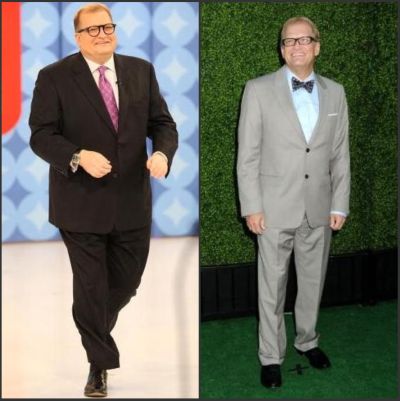In this image, we see two side-by-side photographs of Drew Carey, creating a before-and-after impression. The left photograph features Drew Carey when he was heavier, dressed in a black suit with a white button-down shirt and a pink tie. He is also wearing rounded black glasses. The background suggests he is on the stage of The Price is Right, adorned with a decorative pattern of circles containing diamonds and a red stripe in the upper left corner. In contrast, the right photograph depicts a slimmer Drew Carey in a gray suit with a white button-down shirt and a black bow tie, sporting black shoes. He stands on a green AstroTurf carpet marked with a small 'X' between his feet. Behind him, the backdrop looks like a wall covered in fake green leaves, with a black border running along the bottom. In both images, Drew Carey appears happy and smiling.